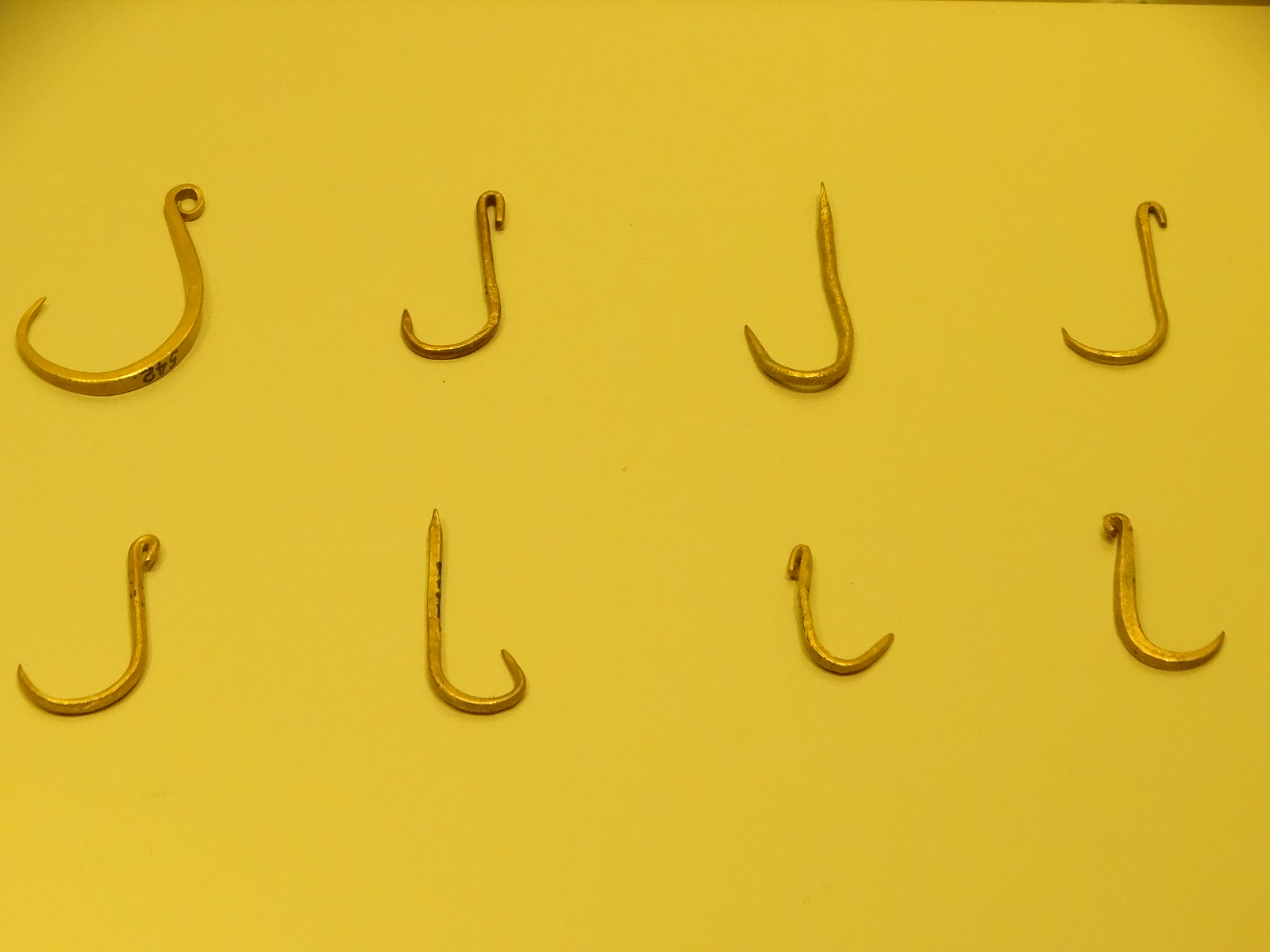The image features a detailed and artistically arranged assembly of eight bronze or gold-colored hooks set against a dark yellow background. The hooks are distributed evenly in two rows of four. The upper left hook is notable for having the number "542" written on its base, characterized by its shape akin to a fishhook, complete with an eye at the top for tying a fishing line. Each subsequent hook on the top row varies slightly: the second is smaller and narrower with a hooked top, the third has points at both ends and resembles a 'J,' and the fourth is J-shaped with an additional small hook at the top.

On the bottom row, the first hook mirrors the top left with its fishhook shape and eye at the top. The second is a backwards 'J' featuring pointed ends, while the third is a smaller, shallow, backwards 'J' with a hooked top. The final hook is another backwards 'J' with a hook on the upper end. The meticulous depiction of these hooks, varying in completeness and form, suggests an artistic exploration of their structural simplicity and functionality.